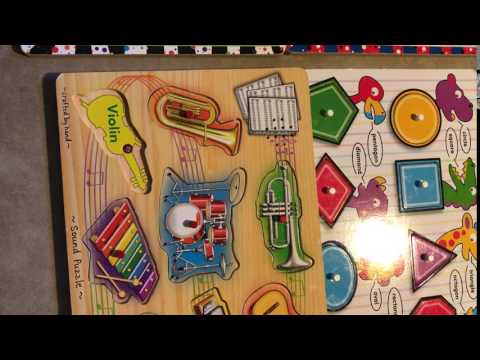The image is a photograph of two vintage wooden puzzle boards designed for toddlers, set against a gray floor. The photograph is bordered by a thin black horizontal line at the top and bottom, giving it an old-fashioned look. The puzzle on the right, which is rotated sideways, features different musical instruments such as a violin, a trumpet, a trombone, a drum set, and a colorful rainbow xylophone, each piece equipped with small red knobs for easy handling by little fingers. The left puzzle showcases basic shapes—circle, square, triangle, trapezoid, oval—each paired with cartoon animal characters. The pieces are brightly colored and designed to be lifted out and matched back into their corresponding cutouts on the board, making them engaging learning tools for young children.